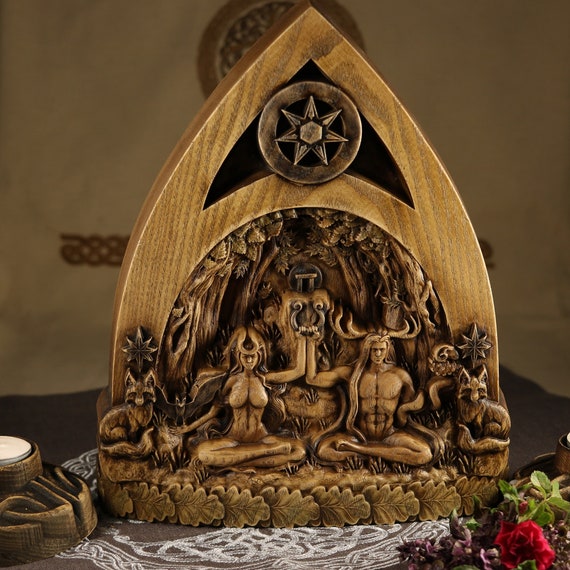This detailed wooden carving depicts a male and a female figure sitting nude with crossed legs, each holding up a harp-like, horseshoe-shaped object. The man, with long hair and horns on his head, has his right arm bent at a 90-degree angle. The woman, whose wavy hair is adorned with a headdress, mirrors his pose with her left arm bent similarly. Flanking the figures, foxes nestle within a wooded scene replete with intricately carved leaves and tree trunks. The top of the sculpture features an arc or a circle, punctuated by a six- or seven-pointed star. This wooden creation, reminiscent of a spear tip in its pointed upper shape, is positioned over a white sewn image set against a grey cloth, decorated with flowers. Flanking this arrangement, candle bottles sit on either side, all in front of a brown tin wall, enhancing the rustic aesthetic of the display.